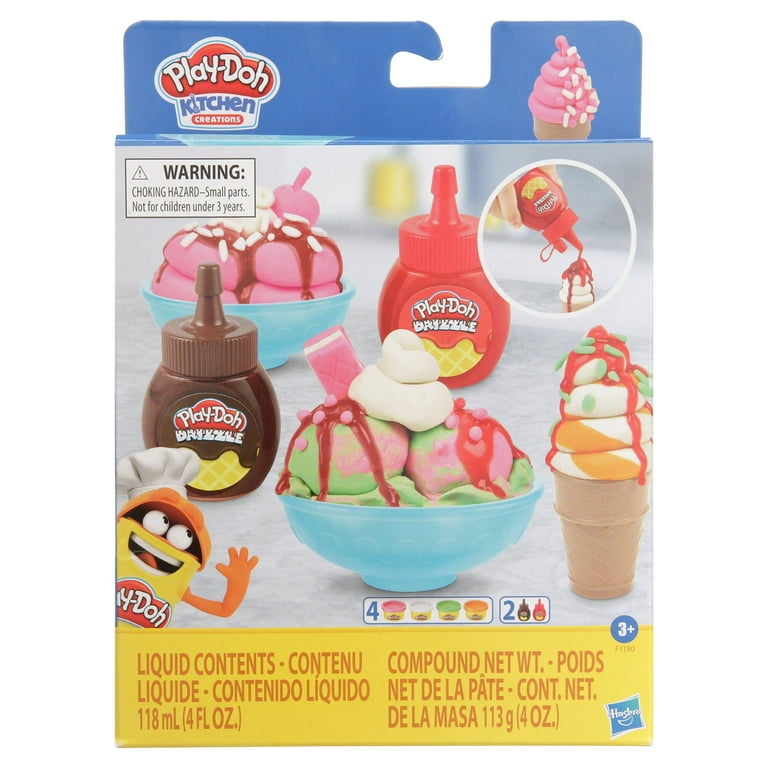The packaging of the Play-Doh Kitchen Creations set is prominently displayed, facing forward toward the camera. The top of the box is blue and features a hook for hanging on store shelves. The top left corner clearly displays the "Play-Doh Kitchen Creations" logo. To the top right of the box, an illustration of a vanilla cupcake with pink icing and sprinkles is shown. Below that, there's a white cupcake base and red frosting with "Play-Doh" written in white letters on the red frosting, and "kitchen" in blue underneath.

The main image on the front of the box showcases various Play-Doh desserts, emphasizing a playful cooking theme. A blue bowl filled with green and pink Play-Doh ice cream topped with white frosting and a pink spoon stands out in the center. Behind it, another bowl contains pink Play-Doh ice cream with chocolate sauce and white sprinkles. Additionally, there are red and brown Play-Doh drizzle bottles depicted, representing strawberry and chocolate flavors respectively.

On the left side of the box, there's a cheerful yellow Play-Doh character sporting a chef’s hat and waving, adding a fun element to the packaging. An ice cream cone featuring white, orange, and green Play-Doh swirled together, possibly with caramel sauce on top, is also pictured. A hand is shown pouring Play-Doh drizzle over the desserts, suggesting interactive play.

Important details such as a warning label indicating the product is a choking hazard and not suitable for children under 3 years old are clearly visible. The bottom left corner of the box includes additional information about the contents and weights, which specify liquid contents and a compound net weight of 113 grams or four fluid ounces. The packaging successfully presents the engaging and creative possibilities offered by the Play-Doh Kitchen Creations set.